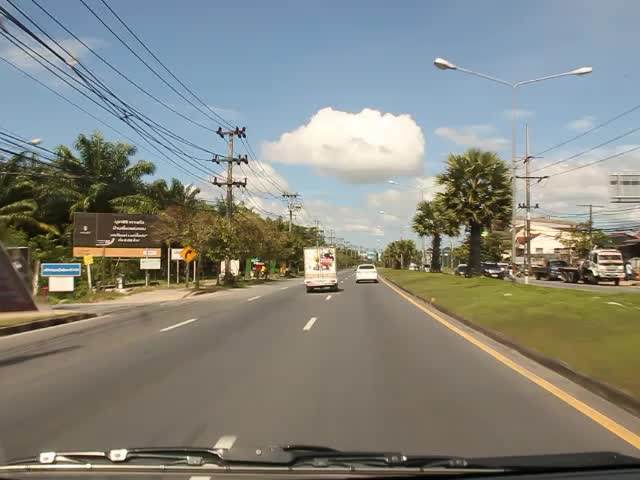This daytime photograph, taken from within a moving vehicle on a three-lane thruway, captures a bright and sunny scene. The sky is a clear blue, adorned with large, fluffy white clouds. Palm trees line the sides of the road, adding a tropical touch to the landscape. Dual streetlamps arch over the thruway and extend into a parking lot visible in the distance on the opposite side of the median. Numerous telephone lines and poles are aligned along both sides of the road. Ahead of the vehicle, there is a white economy car and a cube truck, both traveling in the same direction. Several billboards are also present, though their messages are not legible. The overall scene depicts a leisurely drive on a well-maintained thruway, under a picturesque sky.